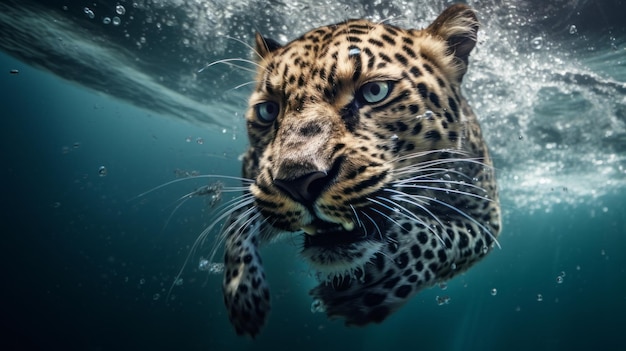This image features an awe-inspiring close-up of a leopard's face as it swims underwater, captured just moments after it dove in. The leopard's wide-open, green eyes with black pupils are riveting, fixed intently on something unseen in the murky depths. Whiskers flare out around a slightly snarled mouth, revealing its bottom canine teeth. Its front paws paddle furiously beneath its chin, creating a dynamic scene. The water, tinted in dark shades of blue and gray, is still turbulent from the splash of the leopard’s entry, with bubbles lingering around its streamlined body. This image, curiously lifelike yet almost surreal, borders on the photorealistic quality of an AI-generated artwork.